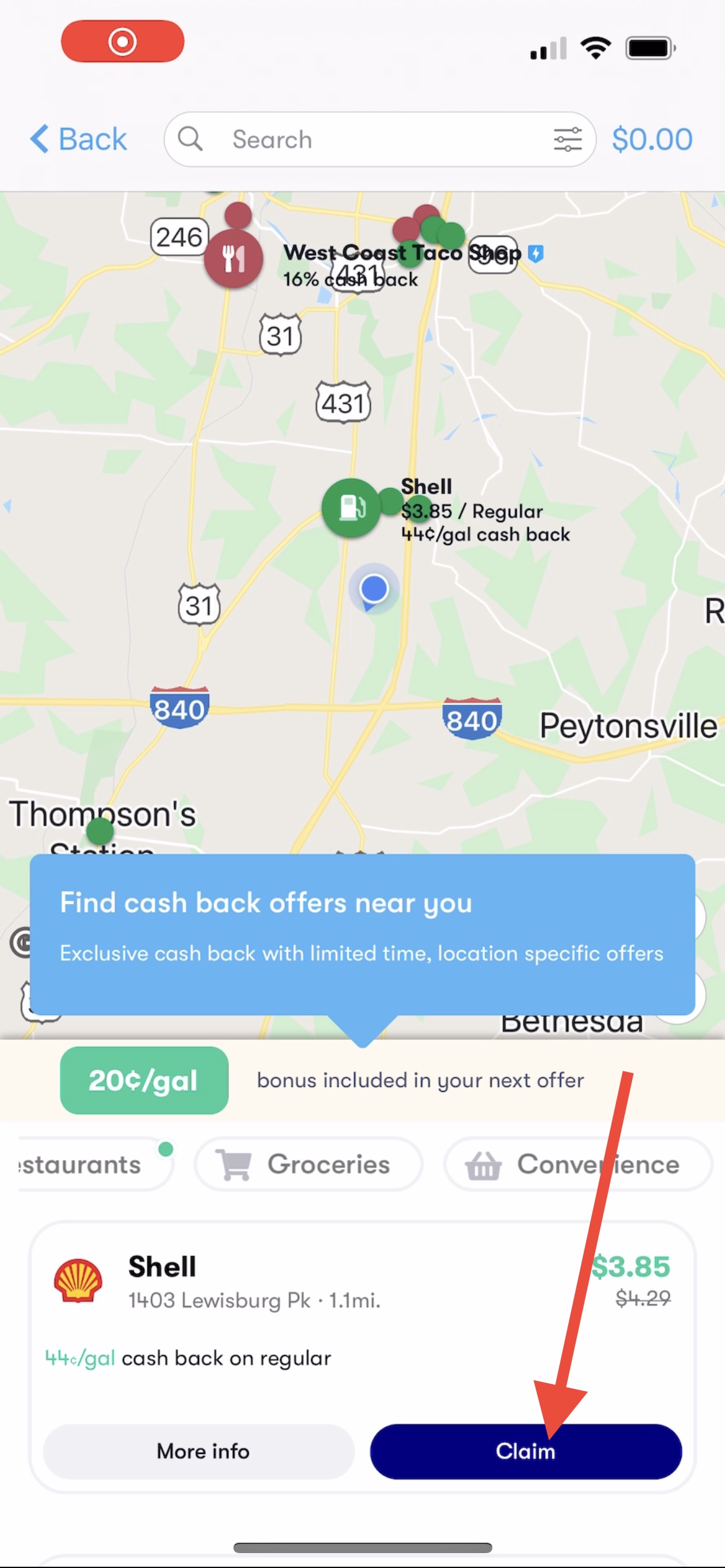The image appears to be a screenshot from a mobile app with a user interface designed for finding and claiming cash back offers. 

At the very top left corner, there's a red rectangular shape with curved edges, featuring a white and red target icon in its center. Next to it, signal strength bars, a Wi-Fi symbol, and a battery icon are displayed.

Beneath this top bar, a blue arrow pointing to the left reads "Back." To the right of this, there is a search bar. Even further right, a blue dollar sign icon indicates "$0.00."

Below this row, a map is shown. Specific locations on the map include "West Coast Tacos," a gas station labeled "Shell," and the cities "Patonsville" and "Thompson Station" near the bottom. Highways 840, 31, 431, and 246 are also visible.

Covering the bottom portion of the map is a blue pop-up banner that reads, "Find cash back offers near you. Exclusive cash back with limited time, location-specific offers." Below this message, there's a green rectangle indicating "20¢ a gallon bonus included in your next offer."

Continuing downward, there are three smaller rectangular buttons labeled "Restaurants," "Groceries," and "Convenience." Beneath these, a larger rectangular section presents details about a nearby Shell gas station at "1403 Lewisburg Park," 1.1 miles away, offering "44¢ a gallon cash back on regular." Prices listed are $3.85, with $4.29 crossed out. A prominent red arrow points to a dark blue "Claim" button, while to its left, there is a light gray "More Info" button.